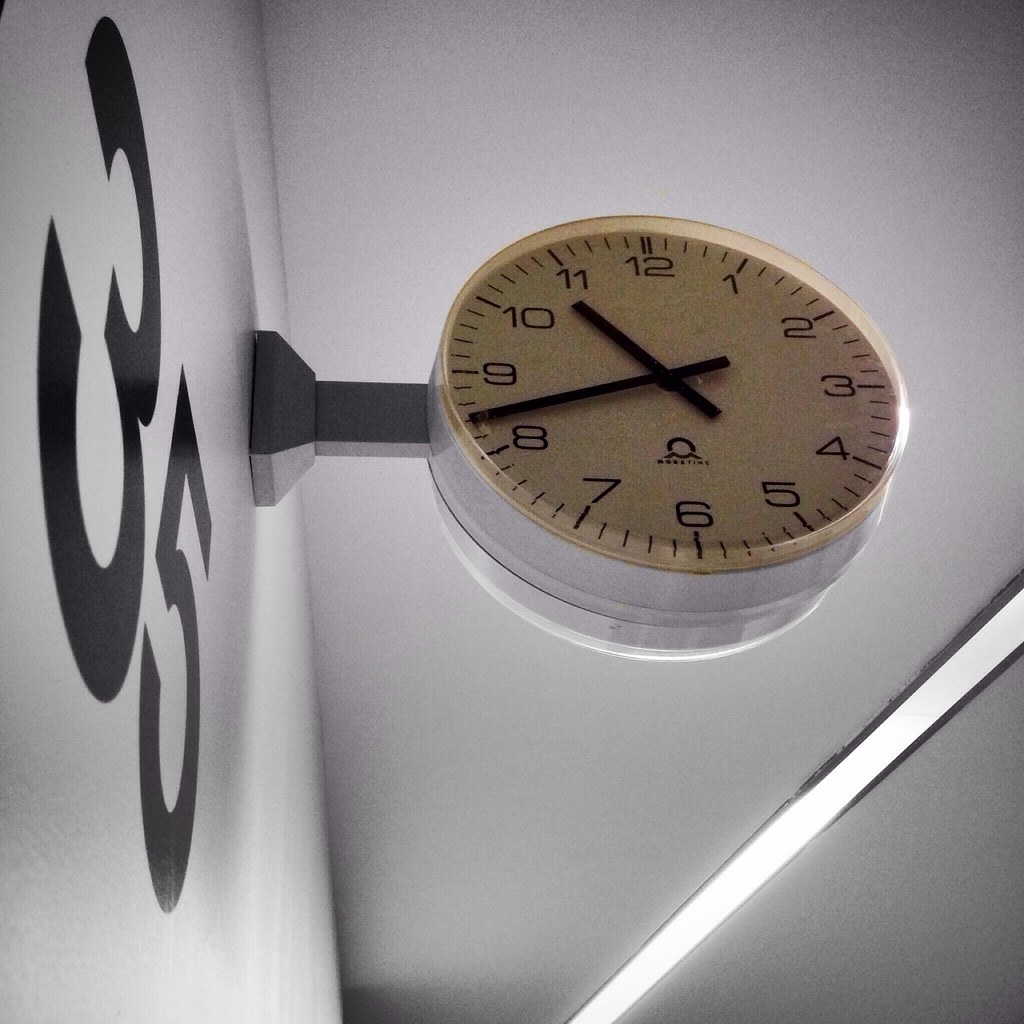The image features a wall-mounted clock centered prominently on a white wall. The clock itself is circular, with a mount that is a stark black, providing a sharp contrast against the wall. The face of the clock is in a yellowish tan hue, with black hands and numbers that strikingly stand out. Notably, the numbers on the clock are arranged in a counterclockwise fashion, adding an element of peculiarity to its design. To the left of the clock, the number "35" is clearly written in black on the wall. The ceiling above is also white, maintaining the stark simplicity of the room’s color palette. On the bottom right of the image, a line of light in white adds an interesting touch to the composition, subtly illuminating the scene.